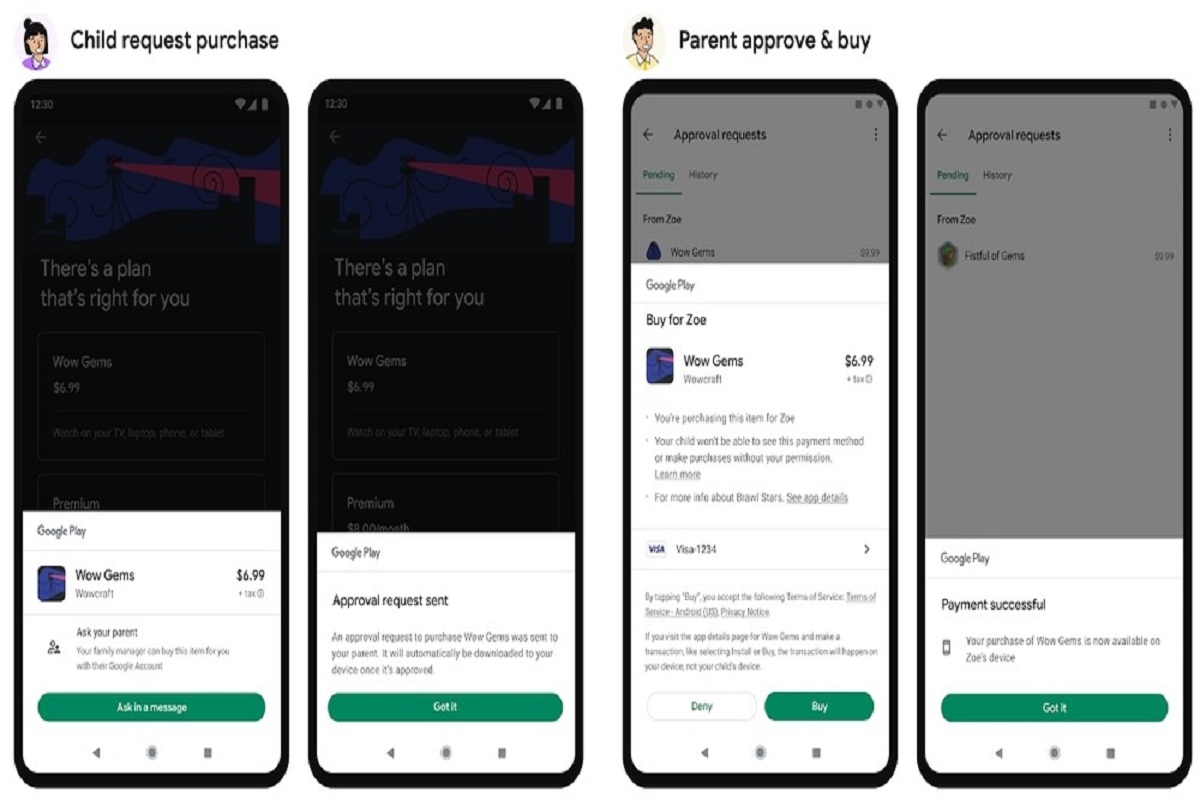In the image, four smartphones are arranged side by side to illustrate a child purchase request and parental approval system. The first two phones are captioned "Child Request Purchase," while the subsequent two are under the title "Parent Approve and Buy." This system highlights how these phones can be utilized to safeguard children.

On the first phone, the screen displays a message saying "There's a plan that's right for you," with a pop-up window for "Wow Gems" from Google Play priced at $6.99. The pop-up box is white with black text and features a green button at the bottom labeled "Ask in a message." 

The second phone shows the child’s purchase request being sent for parental approval.

In the third phone, under the section for parents, the screen shows a tall white box indicating a request from Google Play to "Buy for Zoe: Wow Gems, $6.99." At the bottom of this request, there are two buttons: one for denying the request and another for buying.

Finally, the fourth phone screen announces "Payment successful" indicating that the parent has approved the purchase request.